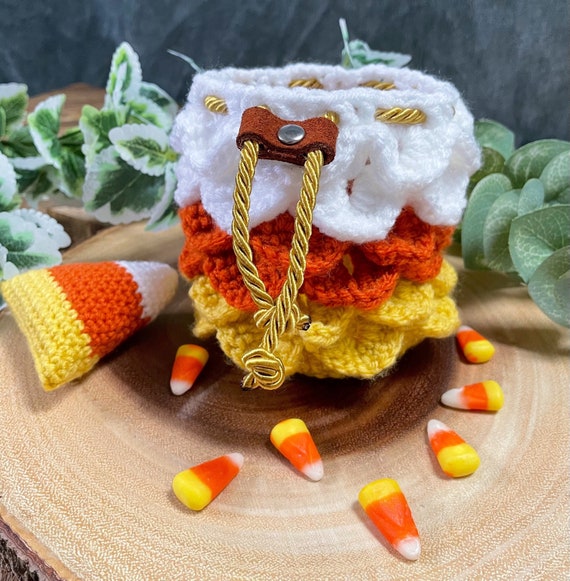In the image, there is a charming, crocheted bag designed to resemble a giant candy corn. The bag, made from yarn, features three distinct layers of color: white at the top, burnt orange in the middle, and yellow ochre at the base. It is cinched closed with a satin gold string adorned with a small brown leather band to secure the ends. The bag is positioned vertically, with its white tip pointing upwards, and it rests on a meticulously varnished, round wooden log slice.

Surrounding the bag are seven real pieces of candy corn, scattered across the wooden surface. To the left of the bag, there is a smaller crocheted candy corn, crafted in the same color scheme—yellow at the bottom, orange in the middle, and white at the top, with its pointed end facing right. The background is decorated with green leaves edged in white, adding a touch of natural charm. The setup is completed with a gray backdrop cloth that elegantly frames the scene, highlighting the festive and autumnal feel of this delightful composition.